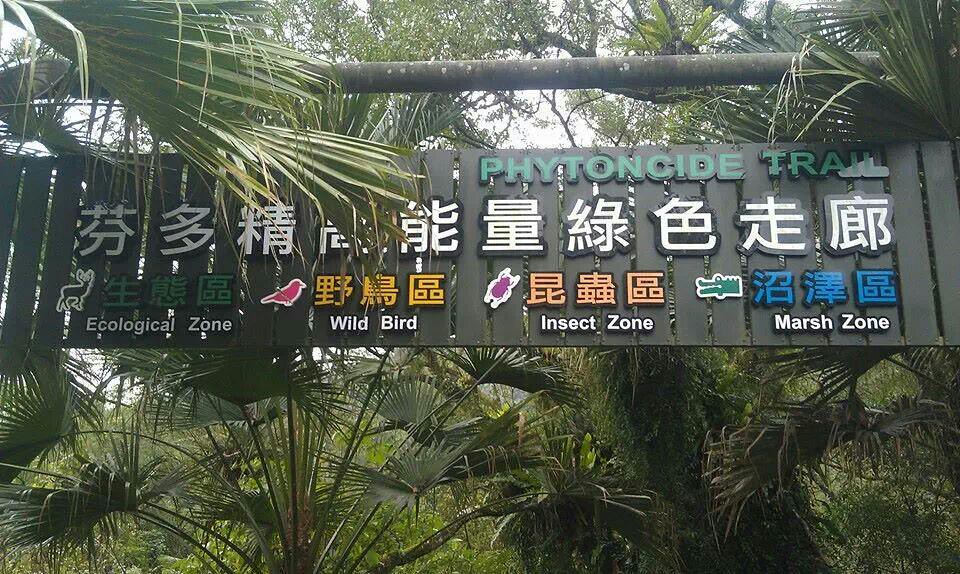In the heart of a lush tropical jungle, a centrally positioned cygnet bird is surrounded by vibrant palm fronds both above and around the sides. The dark green background serves to highlight the informational content on the bird. At the top, "Phytoncide Trail" is prominently labeled in bright green letters, indicating a nature pathway. Below this label, the space is divided into four distinct sections, each accompanied by an icon and presented in both English and likely Chinese text, all in varying colors such as white, pink, yellow, purple, and blue. 

- The first section, "Ecological Zone" is marked by a tree icon.
- The second, "Wild Bird," uses a bird icon.
- The third, named "Insect Zone," features an insect icon.
- The fourth and last section, "Marsh Zone," is represented by a water waves icon.

These sections guide visitors to different areas of interest within the trail. The overall style of the bird and the surrounding elements is both informational and directional, making it clear and accessible for visitors who seek to explore the various themed zones of the trail.